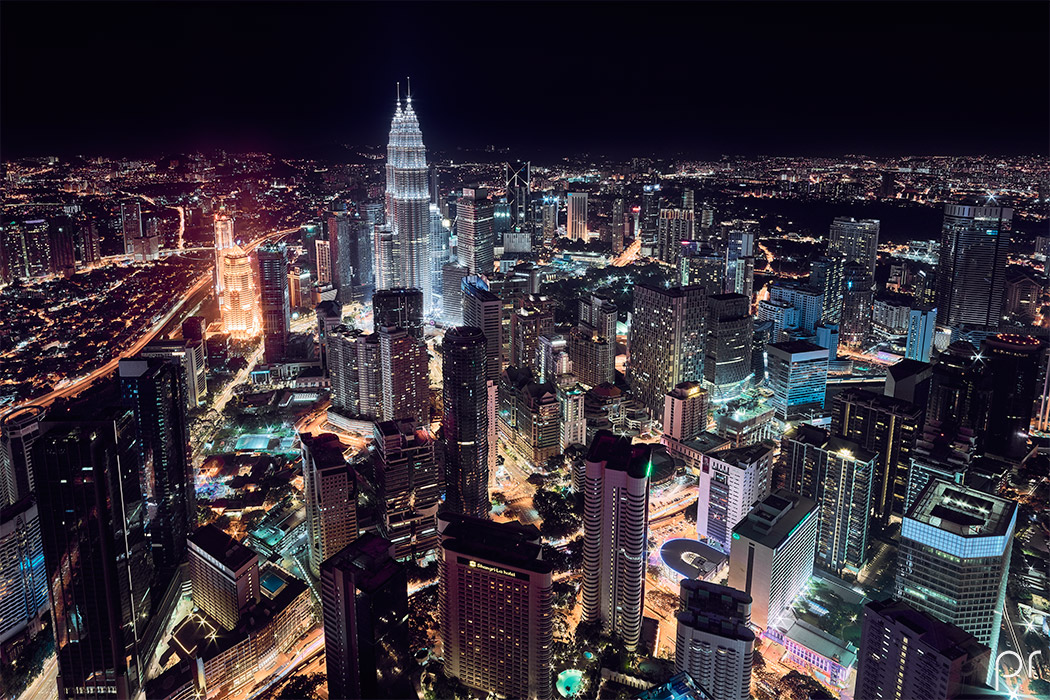This is an awe-inspiring nighttime aerial photograph of a bustling cityscape filled with an array of towering skyscrapers and shorter buildings, all brilliantly illuminated. The black sky serves as a stark backdrop to the vibrant lights emanating from the structures and streets below. The panorama reveals a complex urban landscape with highways teeming with cars whose headlights trace the roads. Notable features include rooftop swimming pools that glow against the dark, and the distinctly lit, architecturally unique tallest buildings in the center – one crowned with dome-like features and another emitting a striking orange hue. The diversity of lights, from bright yellow to deep blue, creates a mesmerizing tapestry of colors. In the bottom right corner, the lowercase letters "PR" are subtly inscribed. Despite the urban density, no people are visible in this stunning scene that captures the city’s electrifying energy from above.